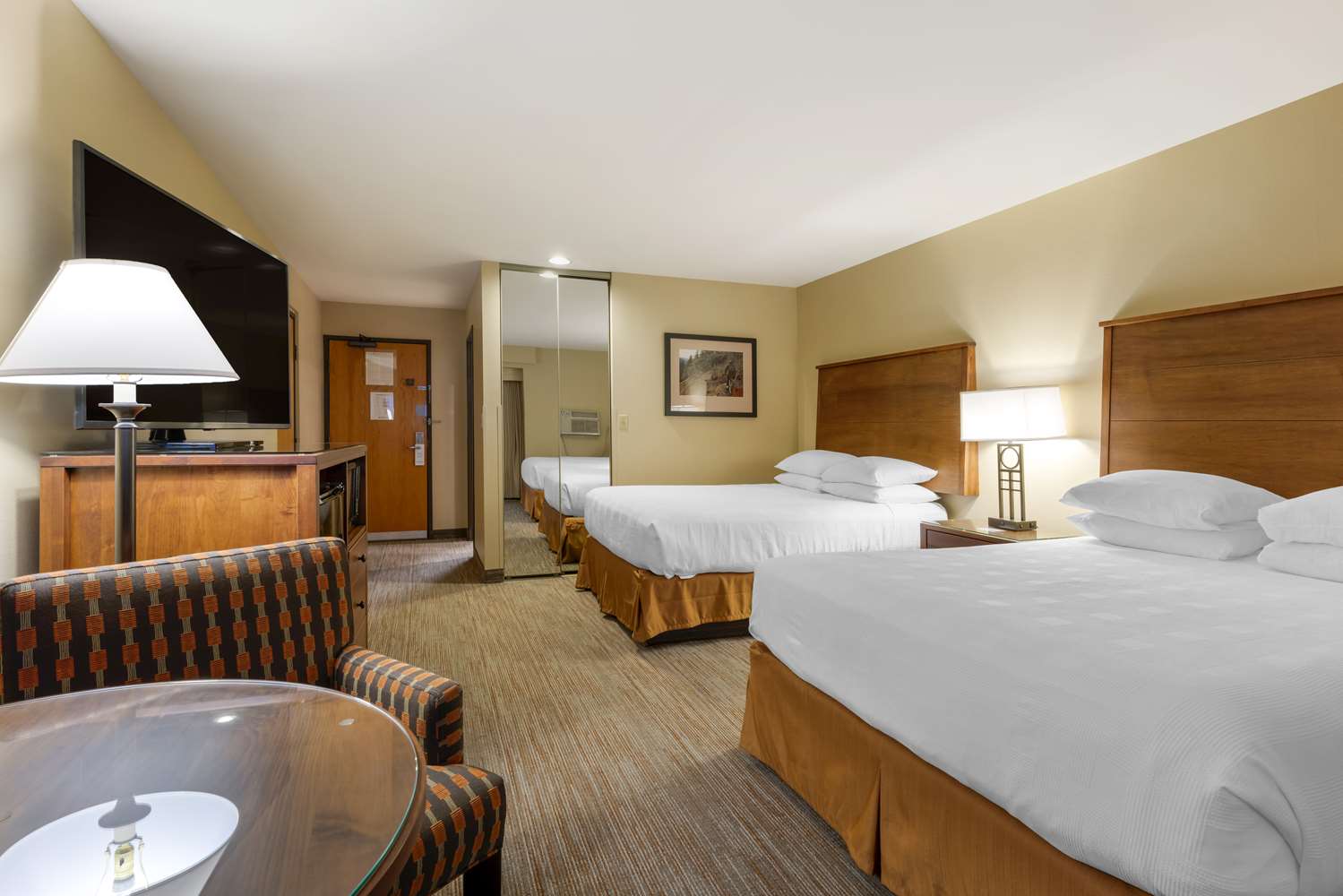This image depicts a typical and somewhat quaint hotel room with a warm color scheme dominated by shades of brown, orange, and tan. The room features two queen-sized beds, each adorned with white bedding, including four white pillows per bed and an almost rust-orange bed skirt. The beds are framed with brown wooden headboards and separated by a nightstand that supports a lit lamp with a white shade and metal base.

On the left-hand side, towards the front, there is a round wooden table topped with glass, paired with an armchair that has a distinctive patterned upholstery in orange, green, and black stripes, combined with red squares. Behind this seating area, a floor lamp with a white shade illuminates the space.

Opposite the beds, there is a wooden dresser with a large flat-screen TV, approximately 55 to 60 inches, positioned atop it. Adjacent to the dresser and further back is the hotel room door, bearing necessary notices and a "Do Not Disturb" tag.

The beige walls host a framed picture and a full-length mirror, reflecting the beds and adding depth to the room. The space is carpeted with light brown flooring, complementing the overall color palette and enhancing the warm, cozy atmosphere.